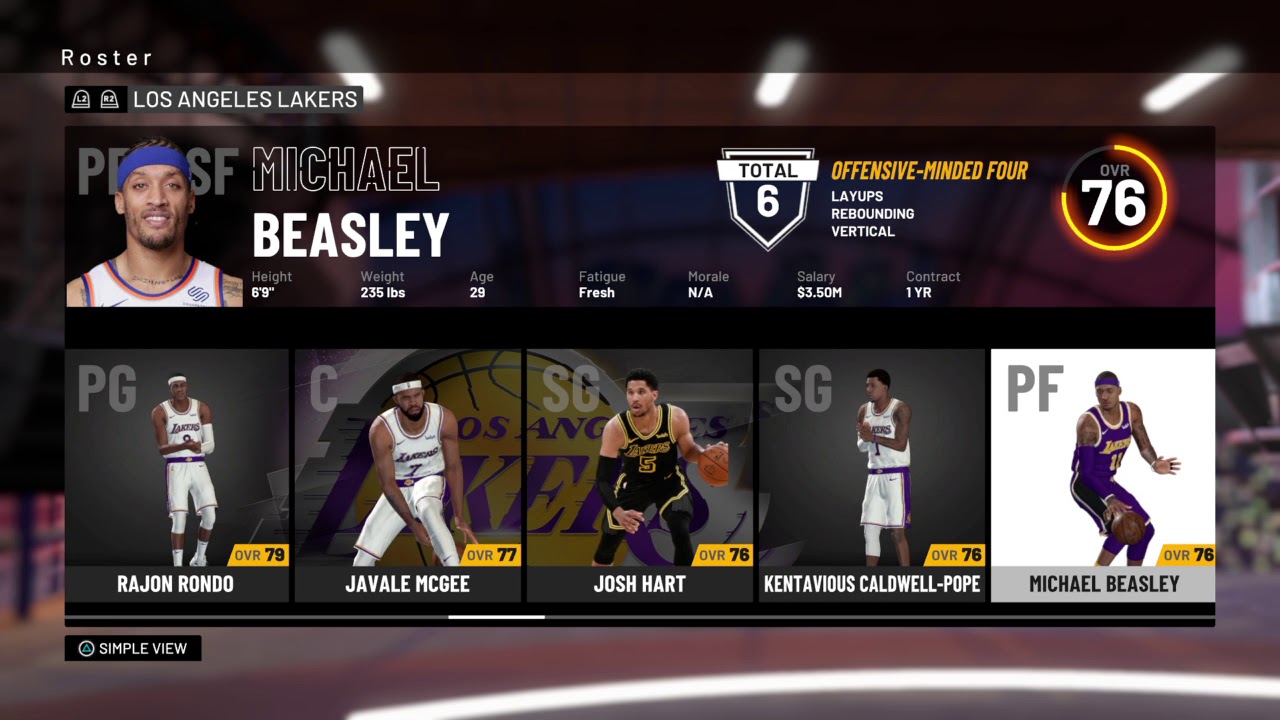This image is a detailed digital screenshot focusing on the Los Angeles Lakers basketball roster. The layout is primarily rectangular and prominently features the team’s comprehensive player information. 

At the very top, the word "Roster" is displayed, directly followed by the team's name, "Los Angeles Lakers," both in bold, eye-catching fonts. Beneath this heading, a dark-colored rectangular section showcases detailed statistics and information about a player. It includes a profile picture of Michael Beasley. 

Adjacent to the image, text provides Beasley's key details: Height - 6'9", Weight - 235 lbs, Age - 29. His fatigue level is labeled as 'fresh', and morale is noted as 'not applicable'. Financial information is also provided, showing a salary of $3.5 million for a one-year contract. This section is marked by an icon reading "Total 6" and "Offensive Minded 4", highlighting specific attributes such as layups, rebounding, and vertical jump.

To the far right of the central rectangle, a circular icon displays an overall rating (OVR) of 76. 

Below the primary section are five smaller images, each showing distinct action shots of players in the midst of a basketball game, emphasizing their active roles in the team. From left to right, the players featured are:
1. Rajon Rondo in a Lakers white uniform.
2. JaVale McGee, also in the white uniform.
3. Josh Hart in a black and yellow uniform.
4. Kentavious Caldwell-Pope in the Lakers white uniform.
5. Michael Beasley finishing off the series as the last player shown in his game gear.

Altogether, the screenshot encapsulates an extensive, detailed overview of the Los Angeles Lakers roster, shedding light on player profiles, attributes, and in-game action shots.